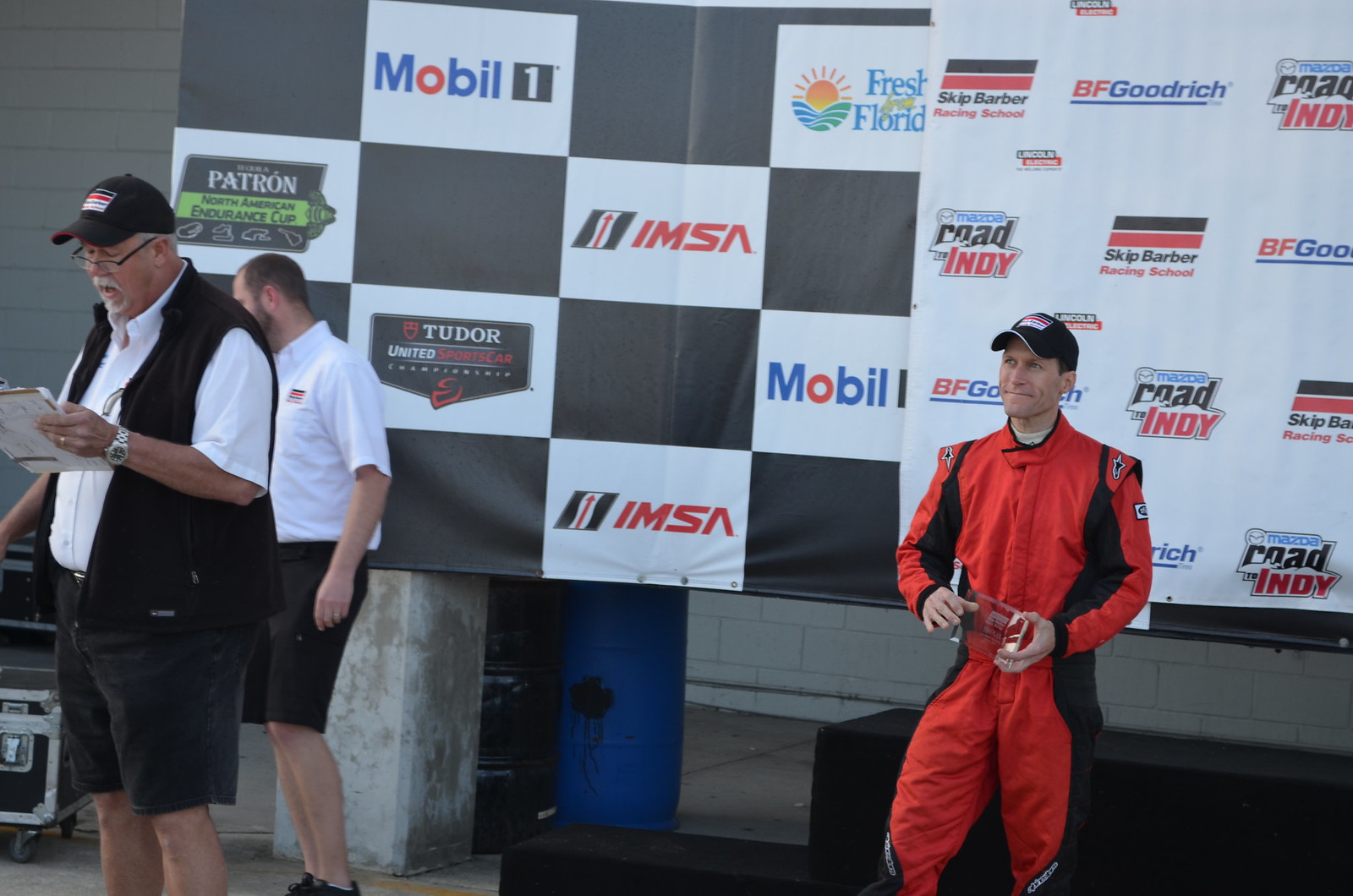This photo appears to have been taken at a racing event, indicated by a prominent banner in the background filled with sponsor logos, including Patron, Mobil One, Tudor United, IMSA, BFGoodrich, Skip Barber Racing School, Mazda, and Fresh from Florida. The banner has a black and white checkered pattern on one side and is predominantly white on the other side.

In the foreground stands a man dressed in a red and black racing suit, complemented by a black, red, and white baseball cap. He is proudly holding a clear trophy, smiling at the camera. To the left, two other men are visible. The man closest to the racer is heavier set, wearing black eyeglasses, a black and white baseball cap, a white button-down shirt, a black vest, and black shorts. He is holding a clipboard and appears to be reading from it. Behind him stands a slightly younger man in a white polo shirt and black shorts, who seems to be waiting for his turn.

The scene captures the conclusion of a race event, highlighting the winning moment and the official proceedings involving the announcement of results.